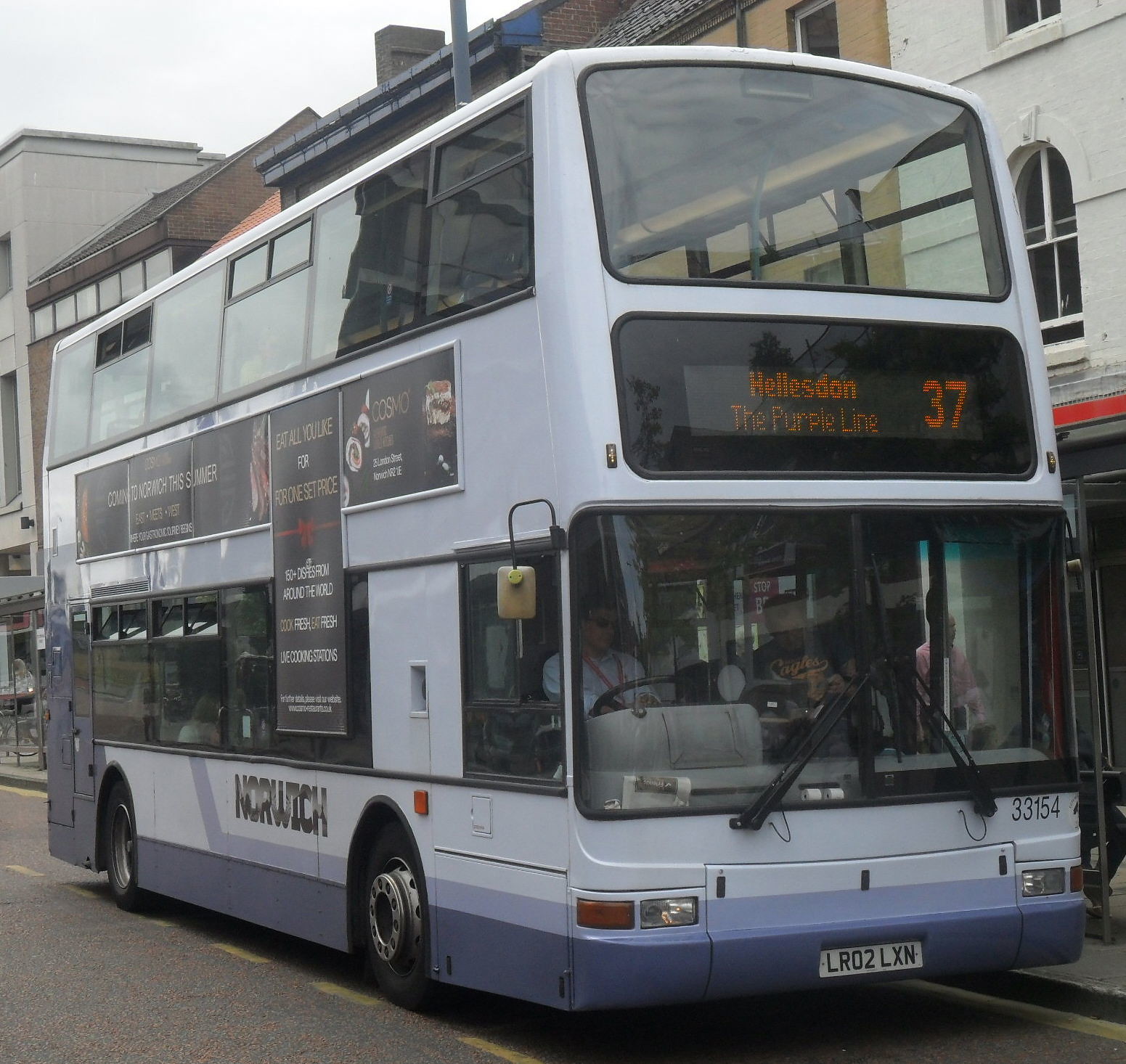A detailed photograph captures a double-decker bus parked at the side of a street, with its doors open and the driver, clad in dark sunglasses and a white shirt, visible at the wheel. The bus is mainly white with a lavender-colored bottom, separated by a light lavender border. It features a digital display in the front windshield, indicating its route as "HELLESDON" on line 37. The side of the bus is adorned with numerous banners and advertisements, though their text remains unreadable from this angle. Notably, there's an advertisement for a restaurant named Cosmo, promising "eat all you like for one set price," with 150+ dishes from around the world, fresh cooking stations, and a note about an upcoming opening in Norwich. Several passengers can be seen inside the bus, which is photographed against a nice blue background.